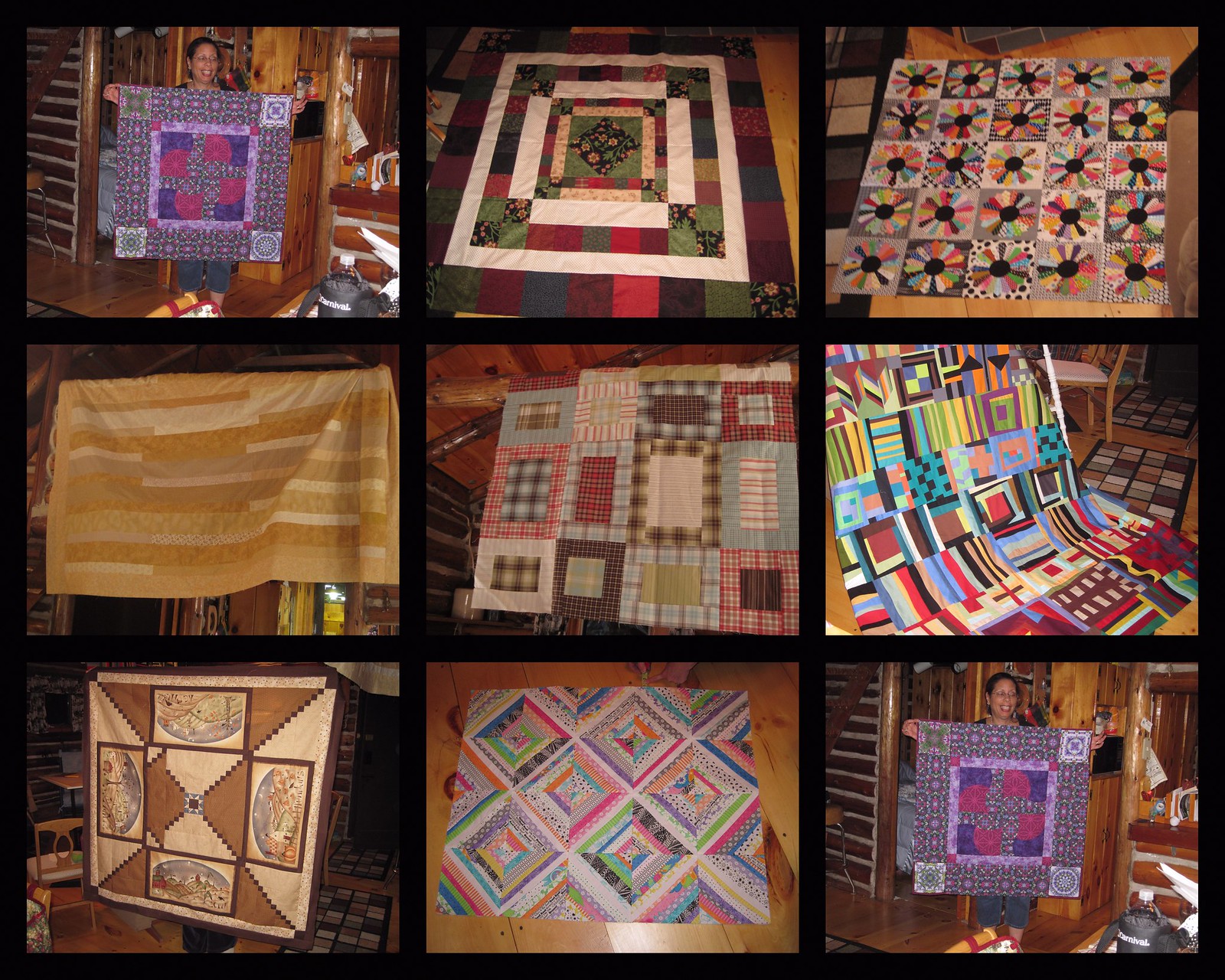This image is a detailed collage of nine different handmade quilts, each uniquely vibrant and artfully stitched. In the top left and bottom right corners, a proud woman is holding a quilt predominantly featuring shades of pink, dark purple, light purple, and a touch of green, arranged in an eclectic pattern. The top middle image displays a quilt with a checkerboard design crafted from red, blue, and green squares outlined in white, interspersed with occasional flowery patterns. Adjacent to it, in the top right, is a quilt with a playful array of circular and petal shapes in rainbow colors. Moving down, the collage includes a yellow quilt composed of horizontal rectangular strips of fabric. There's a mix-match plaid quilt, highlighted by checked patterns, and an eclectic, multi-colored quilt full of vibrant shapes and sprawling designs. Another quilt showcases varied brown triangles meticulously sewn together. This captivating collection captures the artistry and diversity of quilt-making, displaying a rich tapestry of colors, patterns, and designs.